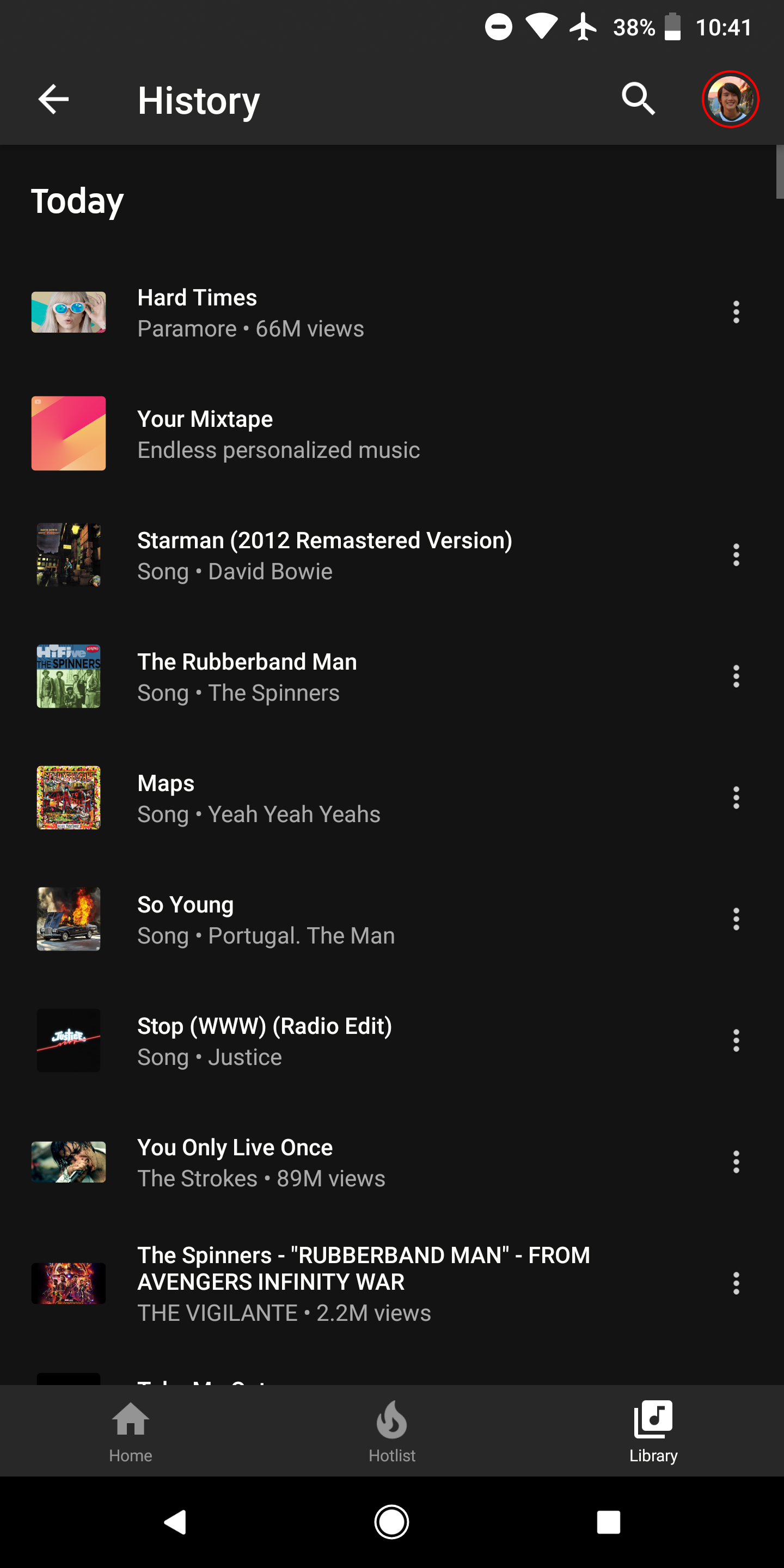Here is an image of a "History" page within a music streaming app, likely resembling Spotify, viewed in a dark mode with a predominantly black background and gray borders. At the top, set in a gray border, there are several notification icons in the upper right corner: a "Do Not Disturb" icon, a Wi-Fi signal icon, and an airplane mode icon. The battery life is shown at 38%, nearly depleted, with the current time displayed as 10:41.

Just below this, a white left-pointing arrow and the word "History" in bold white font are prominently displayed. To the right of this text is a magnifying glass icon for search, a red circle, and a profile picture of a young man with brown hair.

The main content area lists recent listens on a black background. It starts with the heading "Today," followed by:

- "Hard Times" by Paramore with 66 million views
- "Your Mixtape" titled "Endless Personalized Music"
- "Starman" (2012 Remastered Version) by David Bowie
- "The Rubberband Man" by The Spinners
- "Maps" by Yeah Yeah Yeahs
- "So Young" by Portugal. The Man
- "www.radio edit" by Justice
- "You Only Live Once" by The Strokes
- "The Rubberband Man" by The Spinners, noted also for its appearance in "Avengers: Infinity War"
- "The Vigilante" with 2.2 million views

At the bottom of the screen, there is a navigation bar with options labeled "Home," "Hot List," and "Library," with "Library" currently highlighted.